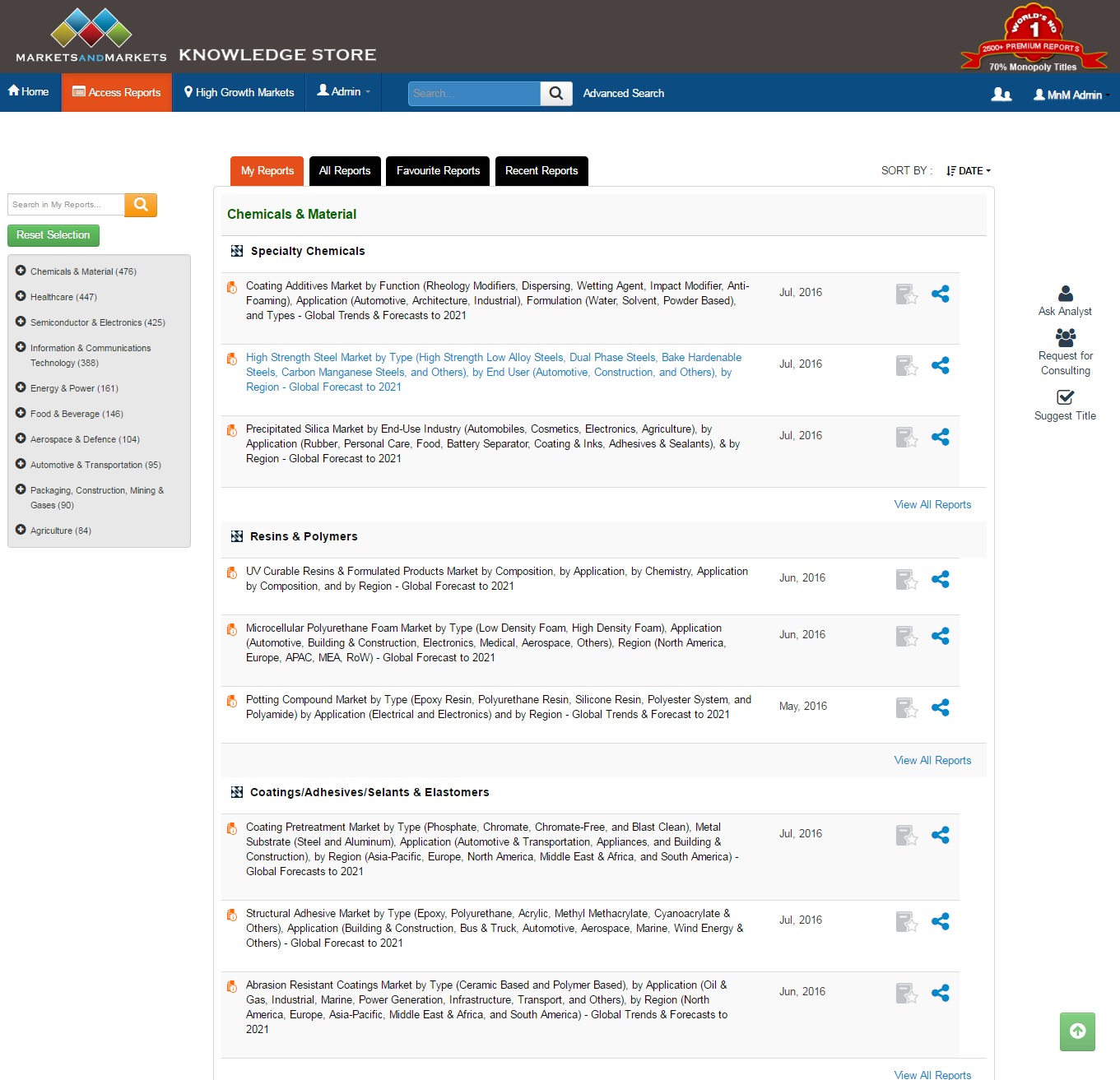Screenshot of the "Markets and Markets" website featuring a clean and well-organized layout. The top section displays a prominent red banner with white text reading "Markets and Markets" on the left and the company's logo, comprised of five squares (two blue squares on top, one yellow square in the center, and two more blue squares to the right), on the right. Adjacent to the logo in the top right corner, there's a red badge with a banner declaring "World's Number One Premium Exports."

Beneath the red banner, a blue navigation bar spans across the page, offering primary navigation options. From left to right, the menu includes: Home, Access Reports, High Growth Markets, an Admin drop-down, a search bar, and a search button. On the far right of the navigation bar are the Profile button and another Admin drop-down selection.

The left sidebar features a secondary search bar at the top, followed by various filter options for refining results. The content area of the website likely contains forms or articles, though it is not depicted in detail in the screenshot.